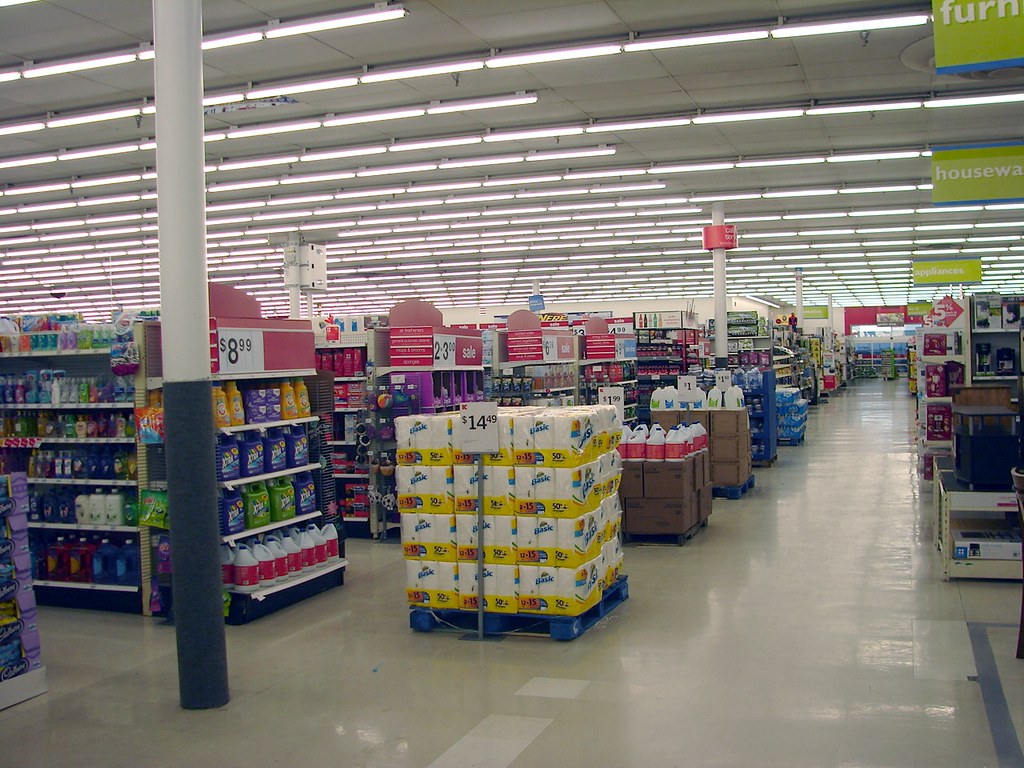This photograph captures a bustling supermarket aisle filled with various products. Prominently featured is a stack of paper products priced at $14.49, alongside pallets of laundry detergent, hand soap, and cases of water. The white tiled floor appears slick and clean, while the ceiling is adorned with fluorescent lights that brightly illuminate the scene. In the center of the aisle stands a steel pillar, half white at the top and gray at the bottom. The aisles, crowded with products, are well-marked by hanging green signs with white fonts and blue stripes, indicating sections like "Housewares," "Appliances," and "Furniture." Cardboard boxes and blue baskets are scattered throughout, holding items for sale. The right side of the image suggests the presence of registers, marked by light yellow ceiling signs, completing the panoramic glimpse of this well-stocked store.